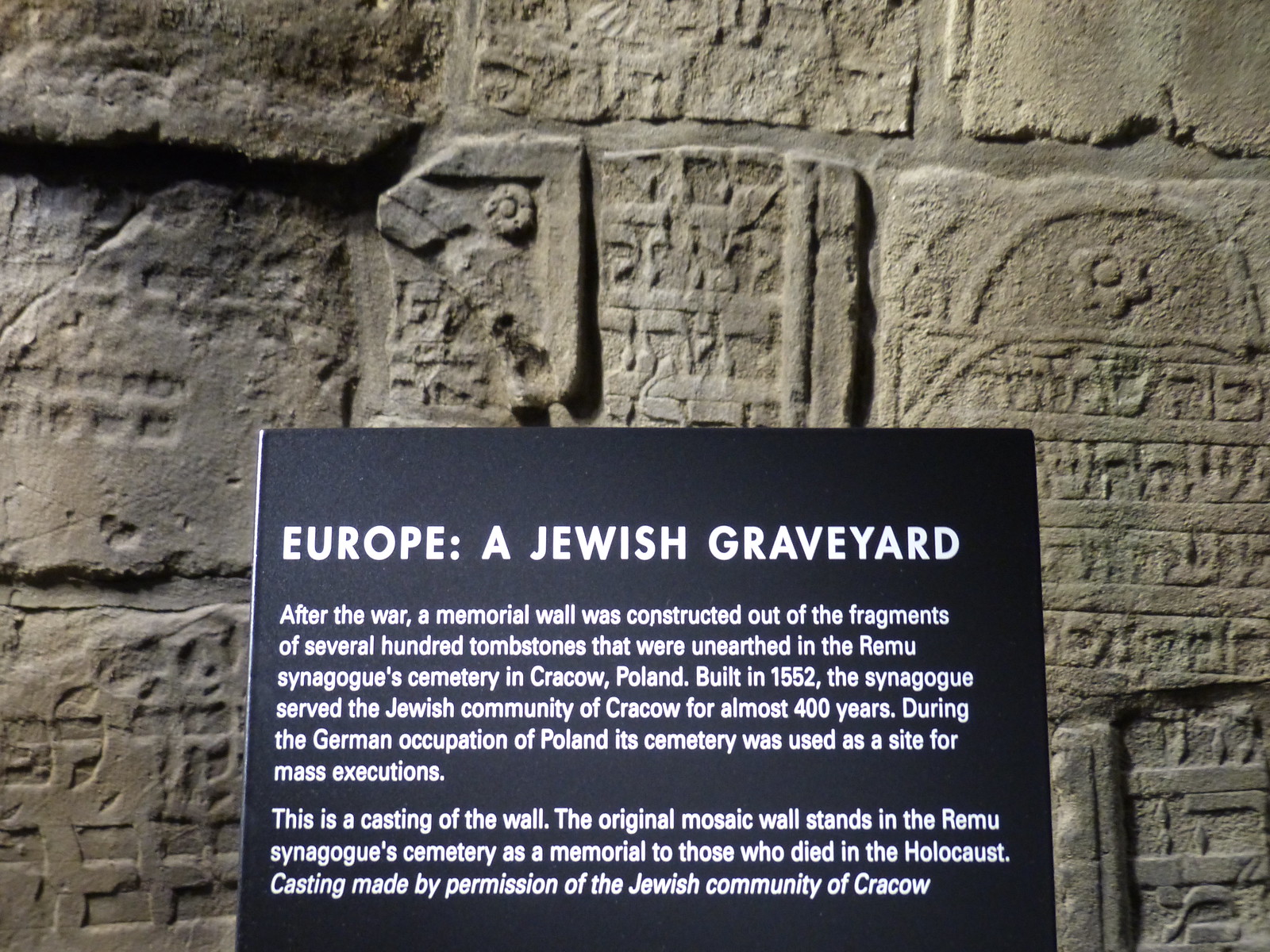The image depicts a black sign with white lettering in front of a stone wall. The headline on the sign, in bold capital letters, reads: "EUROPE: A JEWISH GRAVEYARD." The sign details that after World War II, a memorial wall was constructed from fragments of several hundred unearthed tombstones in the Remu Synagogue Cemetery in Krakow, Poland. This synagogue, built in 1552, served the city's Jewish community for nearly 400 years. The cemetery became a site for mass executions during the German occupation of Poland. The sign explains that the wall in the background is a casting of the original mosaic wall, which still stands in the Remu Synagogue Cemetery as a Holocaust memorial. The casting was made with the permission of Krakow's Jewish community. The stone wall behind the sign, made from various tombstone fragments, displays intricate engravings, including floral patterns and lettered designs, with some pieces shaped like rectangles.